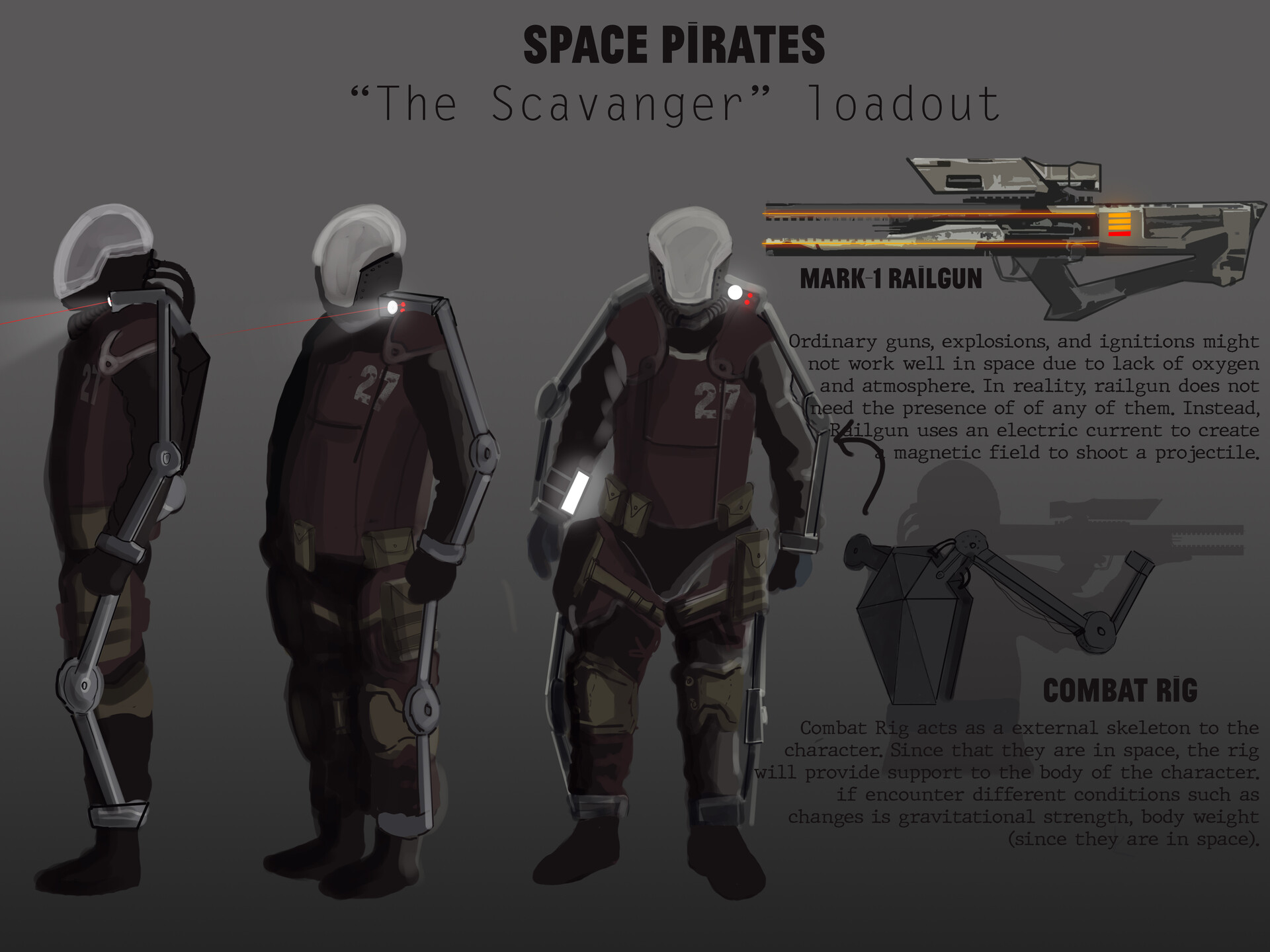The illustration showcases detailed concept art for a character from a series titled "Space Pirates." At the top, in bold, all-capital letters, it reads "SPACE PIRATES," followed by "The Scavenger" in quotes, and beneath it, "Loadout." The character is depicted through three views on the left side: one in profile, one in three-quarters profile, and one facing directly forward. The figure wears a white helmet with three black lines connecting it to the back armor, a dark red vest, and armored trousers. Prominent on the chest is the number "27." Additional features include a flashlight mounted on the right shoulder and a glowing screen on the right wrist.

The character is equipped with an exoskeletal "combat rig" that supports various parts of the body, running along the shoulders, back, arms, and legs. This rig is designed to provide support in different gravitational conditions, essential for space operations.

On the right side of the image is a detailed depiction of the character’s weapon and gear. At the top is a futuristic rifle labeled "Mark 1 Railgun," described as using an electric current to create a magnetic field to fire projectiles, circumventing the limitations of traditional firearms in space's oxygen-free environment. Below the weapon is additional text elaborating on its functionality and an illustration showing the character equipped with the railgun and the combat rig.

The background gradient shifts from light to dark gray, adding depth to the artwork and emphasizing the detailed, futuristic design of "The Scavenger." This comprehensive illustration provides a vivid depiction of the character's equipment and the high-tech, adaptive gear that defines the Space Pirates' aesthetic.